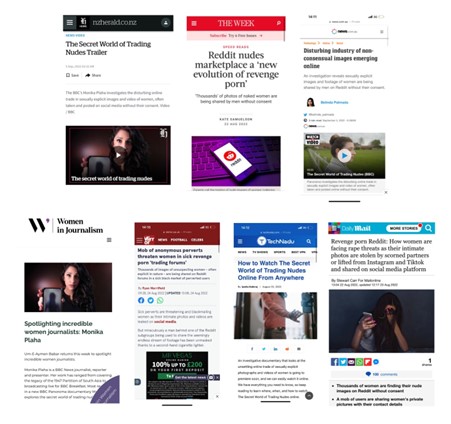This image is a collage of various screenshots taken from a mobile device, all set against a white background. The collage is organized into two rows, with the top row featuring three screenshots and the bottom row displaying four screenshots. 

Starting from the top left, the first screenshot is in black and white and titled "The Secret World of Trading." It appears to focus on a controversial subject, with partial text suggesting it involves the trading of something potentially illicit, possibly "nudes." Centrally located in the collage, the second image is highlighted with the title "Reddit Nudes Marketplace: A New Evolution of Revenge Porn." This central image underscores the disturbing trend of unauthorized sharing of intimate images online. To the right of this, a blurred page with unreadable, small text occupies the third spot in the top row.

In the bottom row, the first screenshot on the left leads with the headline "Women in Journalism," indicating a focus on female professionals in the media industry. Following that, the next image features a distinctive red header, but the detailed content remains ambiguous. The third image hosts a blue and white theme and is titled "How to Watch 'The Secret World of Trading Nudes' Online From Anywhere," implying guidance on accessing prohibited content. Lastly, the fourth image in the bottom row is marked by a green bar at the top, though no additional details are discernible.

Overall, the collage paints a troubling narrative of the digital exploitation of personal images and controversial online behaviors, interspersed with hints of advocacy for female journalists.